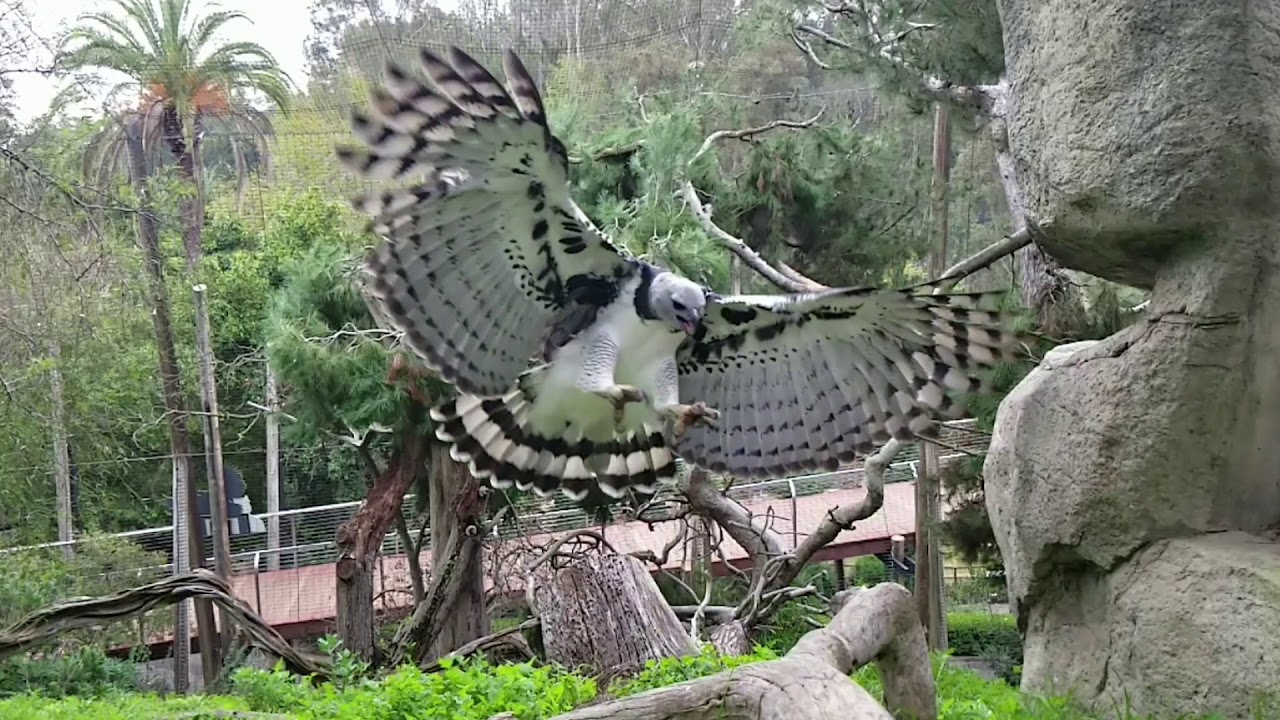The image captures a hawk in mid-flight, positioned dead center and slightly turned towards the camera with its mouth open and its talons outstretched. Its left wing is slightly higher than the right, showcasing the intricate pattern of black stripes on its white underside. The bird's head is gray, adorned with black eyes and a black beak, and it sports a black collar around its neck. The hawk's underbelly is predominantly white, and its tail feathers feature striking black and gray stripes with white tips. Below the bird, a stump is visible in the middle of the frame, alongside a tangle of branches and a distinctive black branch extending from left to right. In the backdrop, there is an array of trees, a red walkway with wooden railings, a stone wall to the right, and a lush green landscape including a palm tree. The photo appears slightly overexposed, rendering the sky a bright white rather than blue.